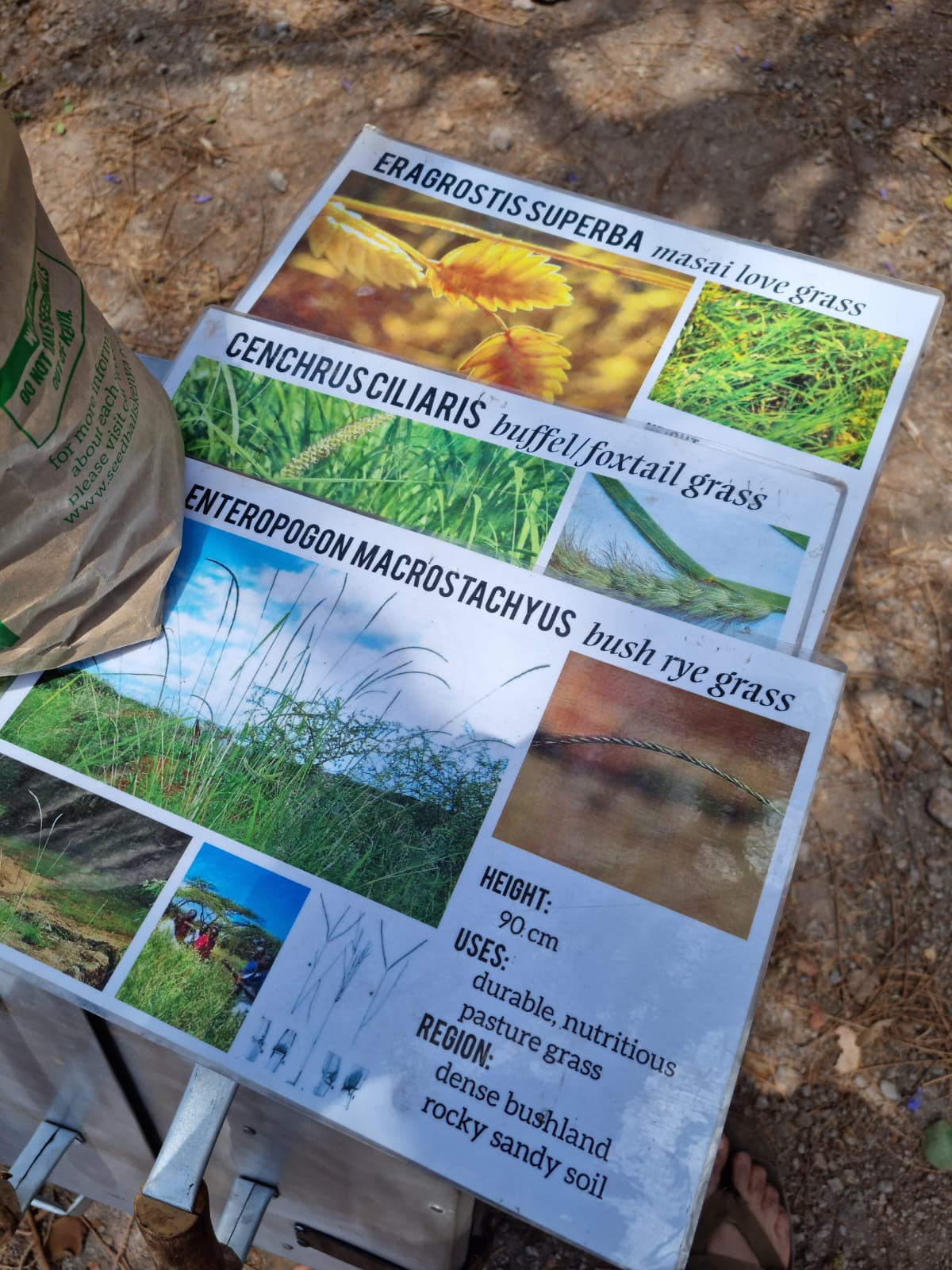The photograph, taken outdoors in portrait orientation, captures three laminated information sheets laid out on a metal box set on a dirt and gravel ground. The sheets are held in place by a brown paper bag on the left side, which reads "for more information about each, please visit seed something.com," implying it may contain seeds. The top sheet is titled "Maasai Love Grass," with the technical name "Eragrostis superba." It features pictures of the grass from various angles. The middle sheet is labeled "Buffalo/Foxtail Grass," technically named "Cenchrus ciliaris," though partially obscured, we can see it similarly includes pictures. The bottom sheet provides details about "Bush Rye Grass," or "Enteropogon macrostachyus." It displays multiple photos of the grass and detailed information, noting its height as 90 centimeters, its use as durable, nutritious pasture grass, and its preferred region of dense bushland with rocky, sandy soil. At the bottom of the image, a sandal can be seen, adding a casual element to the scene.